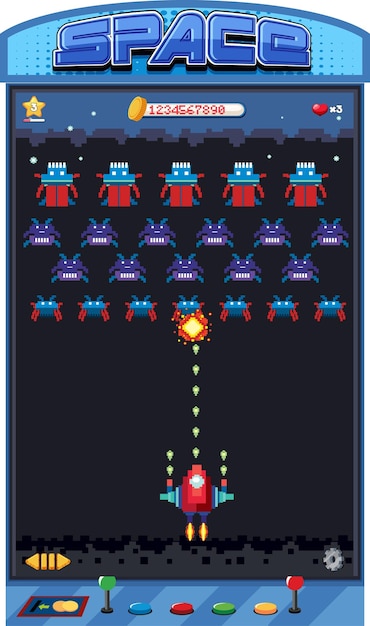The image depicts a vertically oriented, 16-bit graphic design mock-up of an old-school arcade game resembling Space Invaders, titled "Space." The game screen shows a spaceship at the bottom of the screen, shooting bullets upwards toward four rows of evenly spaced alien creatures in various colors: the top row features red aliens with blue faces, the middle two rows have purple aliens, and the bottom row consists of blue aliens with red legs and arms. The game indicates that the player is on level three, has three lives (represented by hearts), and a total score or coin score. The top center of the game screen displays the title "Space" in a gradient of light to dark blue font with a star icon on the left and a sequence of numbers (1, 2, 3, ...) in red, inside a white circular box in the middle. The scene is framed by the arcade cabinet interface below, which includes green and red joysticks, and multicolored buttons (blue, red, green, and yellow), along with other familiar controls like push buttons, pull knobs, toggles, and a coin slot, all contributing to the retro gaming ambiance.